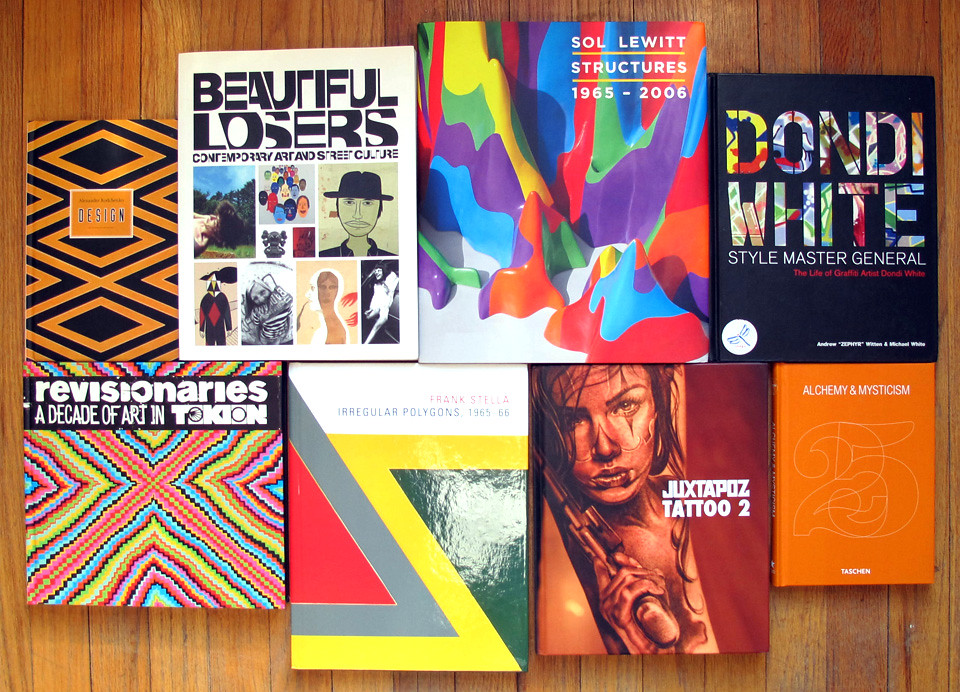The image depicts an artistic arrangement of eight diverse books, meticulously aligned in two rows of four on a vertically laid, medium-toned hardwood floor. The books exhibit varied sizes and themes, unified by their artistic content. From left to right, the top row features: a book with an optical illusion design of alternating black and orange triangles, a white book titled "Beautiful Losers" showcasing contemporary art and street culture, a multicolored book, "Sol LeWitt: Structures 1965-2006," displaying a vibrant array of colors that resemble abstract mountains, and "Donde White: Style Master General," a sleek black book. The bottom row begins with "Revolutionaries: A Decade of Art in Toucan," followed by "Irregular Polygons 1965," a book that’s slightly hard to decipher, "Tattoo II," which highlights intricate tattoo designs, and concluding with "Alchemy and Mysticism," notable for the number 25 on its cover. The photo, captured from above, emphasizes the collection’s visual harmony and artistic diversity.